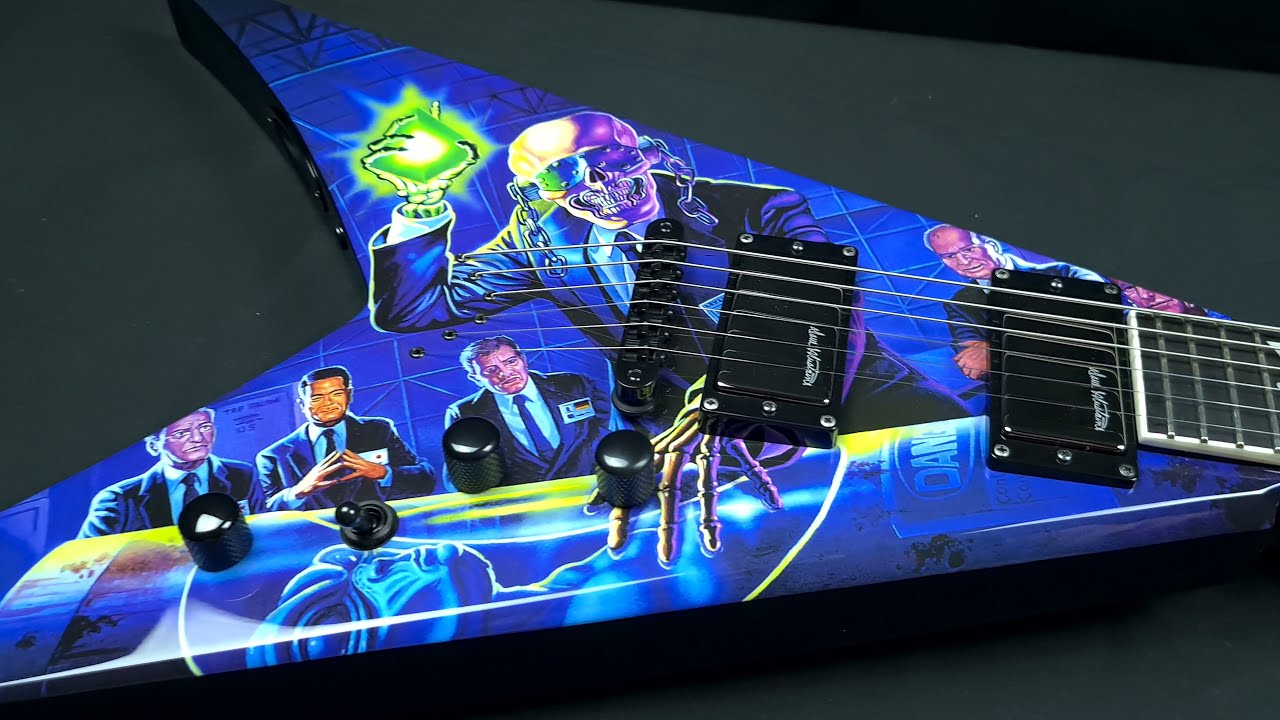This is a detailed close-up photograph of the bottom portion of an angular, Flying V electric guitar adorned with a complex, fantasy-style illustration. The guitar, intended for a right-handed player, is painted in a deep purple-blue hue and is positioned sideways against a dark gray table or black desktop. The illustrated scene on the guitar's surface depicts a dramatic tableau set against a blue background that suggests a warehouse ambiance with scaffolding visible in the distance.

Central to the illustration is a skeleton dressed in a blue business suit, standing over a coffin-like tube labeled "danger" containing an alien life form. The skeleton figure is holding a glowing green diamond aloft in his right hand while his left skeleton hand reaches towards the alien, extending under the guitar strings. Surrounding the alien-containing tube are several businessmen also dressed in suits and ties; three are seated on the left side of the skeleton, looking on intently, while to the right stands another businessman with one more seated beside him. The scene on the guitar evokes themes of extraterrestrial containment and a critical evaluation, reminiscent of an Area 51-like scenario. The photograph captures the oil-painted illustration in vivid color and elaborate detail, blending elements of representational art and fantasy into a striking visual narrative.